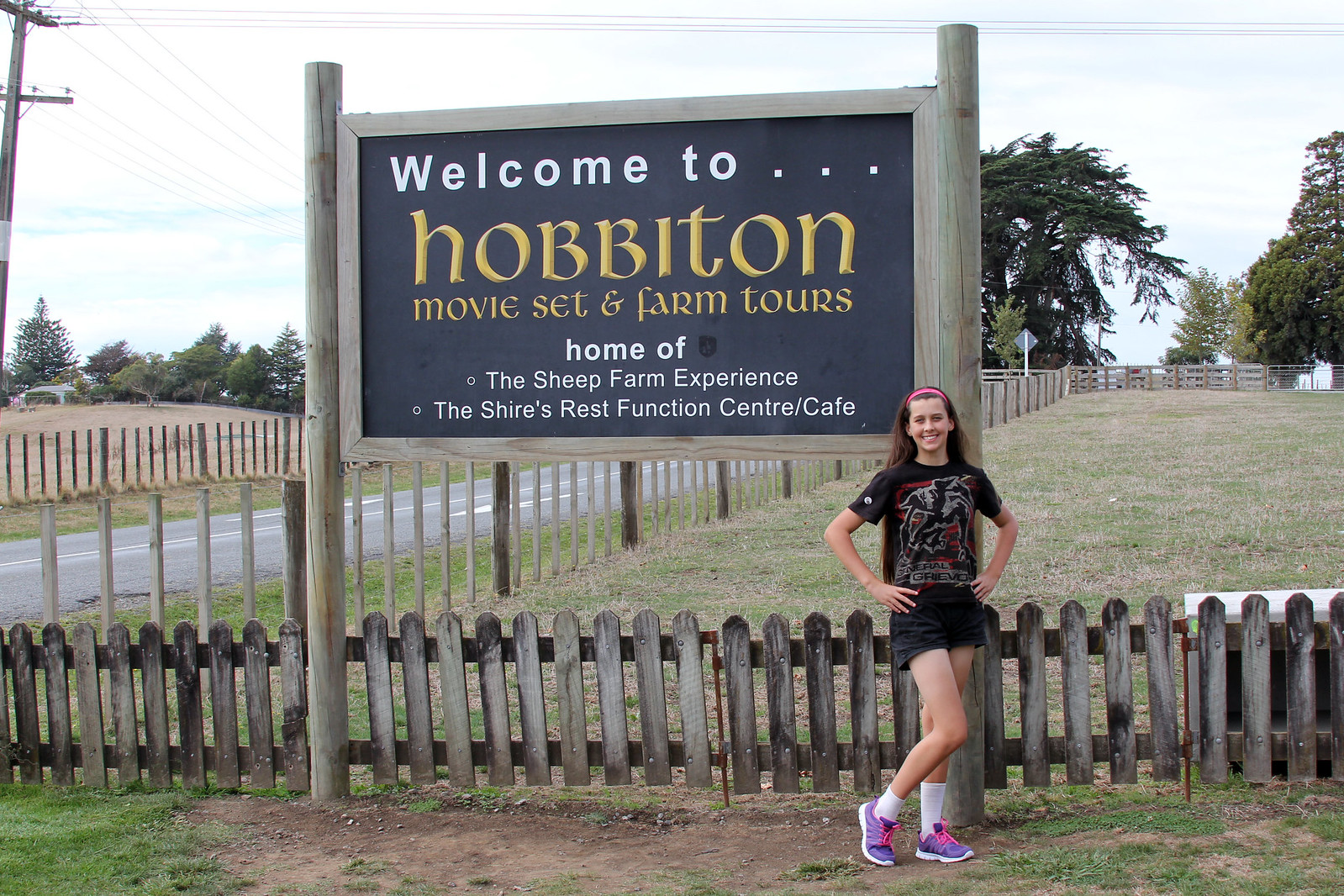In this outdoor daytime photograph, taken in landscape orientation, we see a scenic field framed at the bottom by an aged wooden picket fence, weathered to a gray hue. Directly in front of a post on the right-hand side of the image stands a young Caucasian girl, likely in her mid-teens. She has shoulder-length brown hair, held back by a pink headband, and is smiling warmly. Dressed in a black graphic t-shirt with what appears to be "General Grievous" printed on it, she pairs this with black shorts, white socks, and purple sneakers accented with pink laces. Her hands rest confidently on her waist.

The post behind her holds a sign with a black background and white and gold text. The sign welcomes visitors to "Hobbiton Movie Set and Farm Tours," further detailing amenities such as the "Sheep Farm Experience" and "The Shire’s Rest Function Center/Café." The field behind her stretches into the distance, bordered by further fencing, and interspersed with trees and power lines. To the left of the image, a two-lane road meanders into the horizon, flanked by additional fields and dotted with more trees, beneath a sky that blends white and light blue tones.